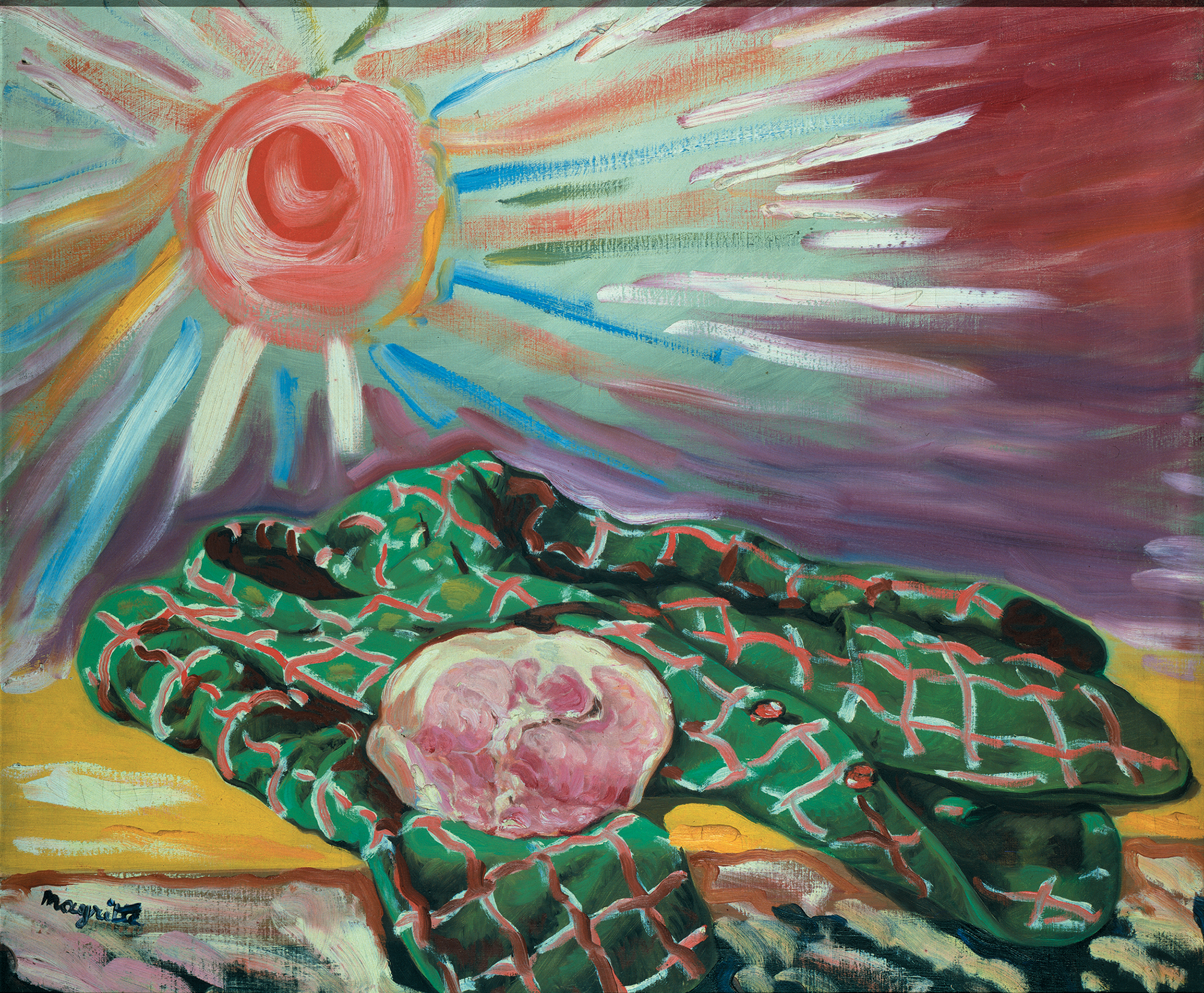The painting is a colorful and expressive work featuring a prominent red circle in the upper left, representing the sun. From the sun emanate varied rays in blue, yellow, white, green, blue, red, and orange, creating a vibrant sky in shades of red and purple. The background is adorned with a spectrum of colors emphasizing nature. In the foreground, there is a horizontal yellow surface, reminiscent of a bench or table. Laying across this surface is a green men's suit jacket with a red windowpane design and red buttons. Atop the jacket rests a reddish hat or beret. The painting is devoid of people, with a small amount of text in the bottom left corner, likely the artist's signature in black font. The composition suggests themes of rebirth or an artistic representation of Earth. White and black marks are visible at the very bottom of the painting, adding to its intricate detail.